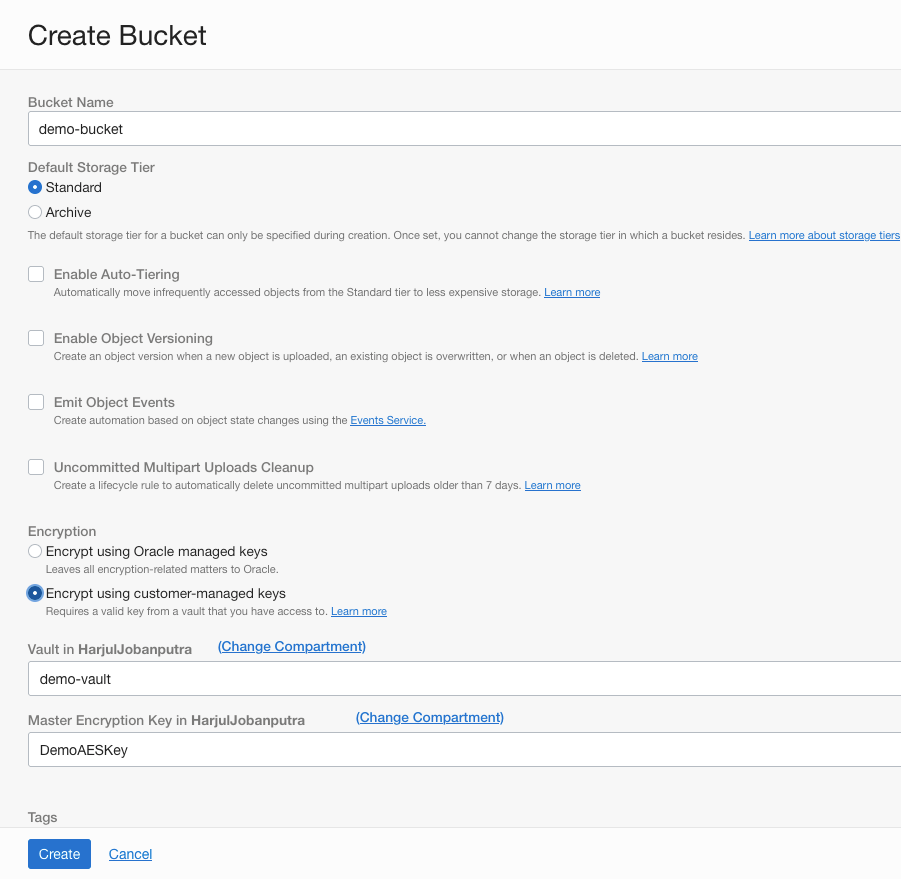In this black-and-white screenshot of a web page, we see the interface for creating a new storage bucket. The header at the top reads "Create Bucket." Below this, there's a section for entering the "Bucket Name," with a writable field labelled "demo bucket."

Following this, there's a section for setting the "Default Storage Tier," where two options are provided: "Standard" and "Archive," with "Standard" being pre-selected. A note clarifies that the default storage tier can only be specified during the bucket's creation and cannot be changed later.

Further down, we encounter options for additional settings: "Enable Auto-Tiering," "Enable Object Versioning," "Emit Object Events," and "Uncommit Multi-Part Uploads Cleanup." 

The next section deals with encryption settings. The first option, "Encrypt using Oracle Managed Keys," is unselected, while the second option, "Encrypt using Customer Managed Keys," is selected. Beneath this, fields are filled in with "Vault in harjuljabanputra" and "Demo Vault." Additionally, the master encryption key is indicated as "Demo AES Key" under the same vault.

At the bottom of the page, a button labelled "Create" awaits to finalize the bucket creation process.